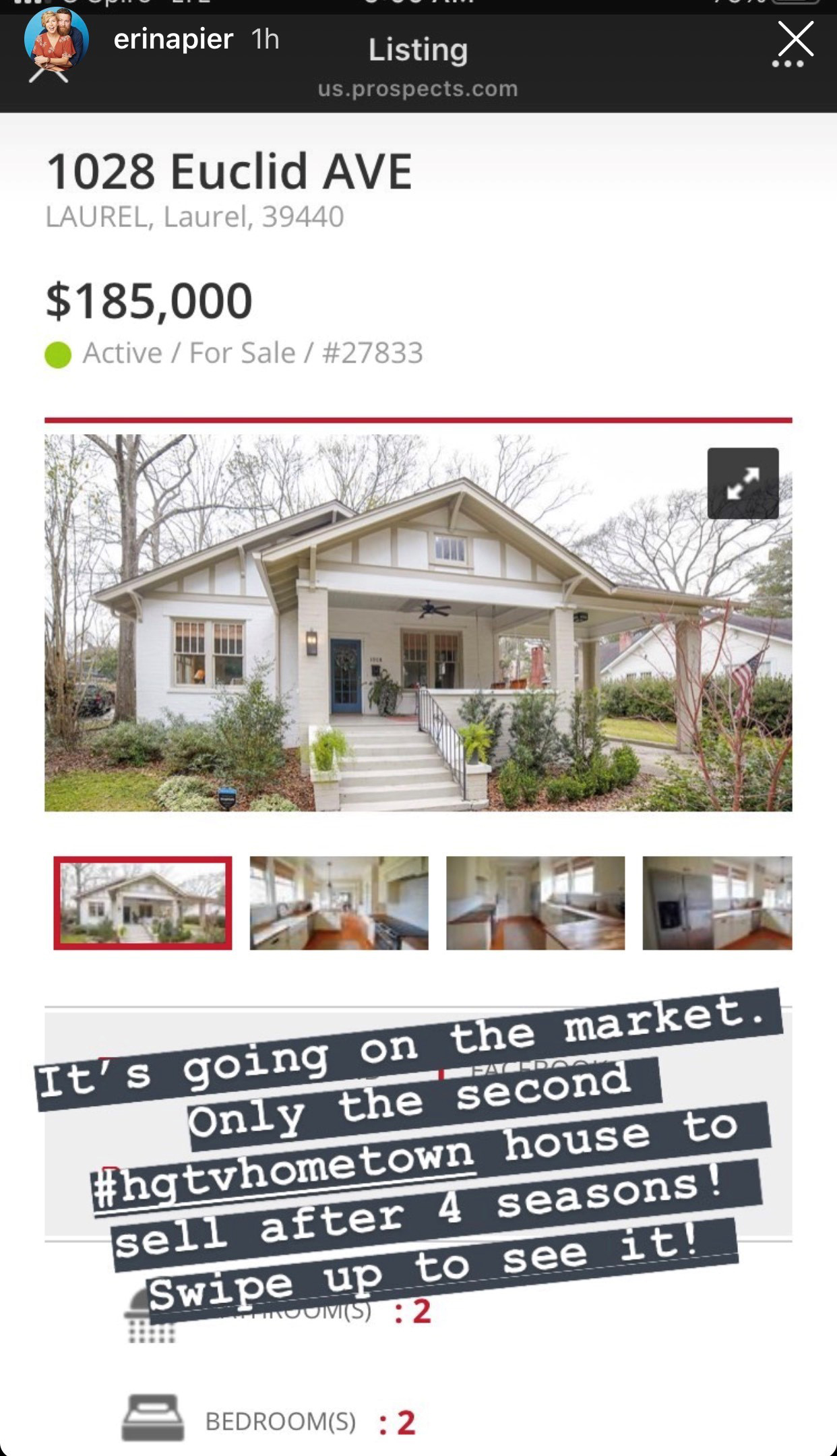Screen capture of a real estate website, likely showcasing a property listing. At the top of the image, there's a black banner displaying the username "Aaron Napier" along with a profile picture of two people embracing. The website URL "listingus.prospects.com" is visible below this banner.

In bold black text, the property address is listed as "1028 Euclid Avenue, Laurel, MS 39440," with an asking price of $185,000. Accompanied by a green dot, the listing status is marked as "Active for Sale," with the listing number "27833."

The featured image is of a white home with stairs leading up to a porch area. The front door is blue and a black ceiling fan is mounted under the porch. Tan trim accentuates the house's features, and green shrubbery along with bare trees can be seen in the surrounding yard. Above this image, there's a thin red line. 

Below the main image, multiple smaller images are shown in a series. The highlighted image is the one previously described. The other images displayed are interior shots, notably the kitchen, which includes white cabinets, a large stainless steel refrigerator, and an orange-toned floor. 

Further down, in bold black and white text, it states, "Going on the market, only the second #HGTVHometown house to sell after four seasons. Swipe up to see it." 

Additional property details are indicated with red icons: "2 Bathrooms" with a showerhead icon and "2 Bedrooms" with a bed icon.